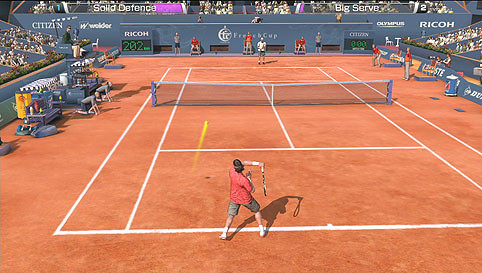This screen grab captures an intense moment from the video game Virtua Tennis. Set on a vibrant orange clay court with crisp white lines, the scene showcases two tennis players mid-match. The net is detailed with blue sections flanking the white tape at the top. In the foreground, a player dressed in a red shirt and gray shorts prepares for a return, holding his racket in his left hand while his right hand is extended forward. His white sneakers blur slightly with motion, hinting at his swift agility.

The opposing player, positioned across the court, sports a white shirt, white hat, blue pants, and black shoes, though his racket is not visible. The backdrop features a prominent blue wall with the brands "Citizen" and a word that appears to be either "Wiedner" or "Wider" displayed. Additionally, the text "Recon" accompanied by the number "202" appears on a digital display, possibly indicating a speed measurement, though its exact relevance is unclear.

The spectators contribute to the game's lively atmosphere. On the right-hand side, a packed crowd watches intently, with two men notably kneeling on the ground—a unique sight in a tennis game. Along the left side, men in red jackets and gray pants, possibly referees, are seated, overseeing the match. More spectators fill the stands that span the back of the court, reinforcing the sense of a high-stakes tournament.